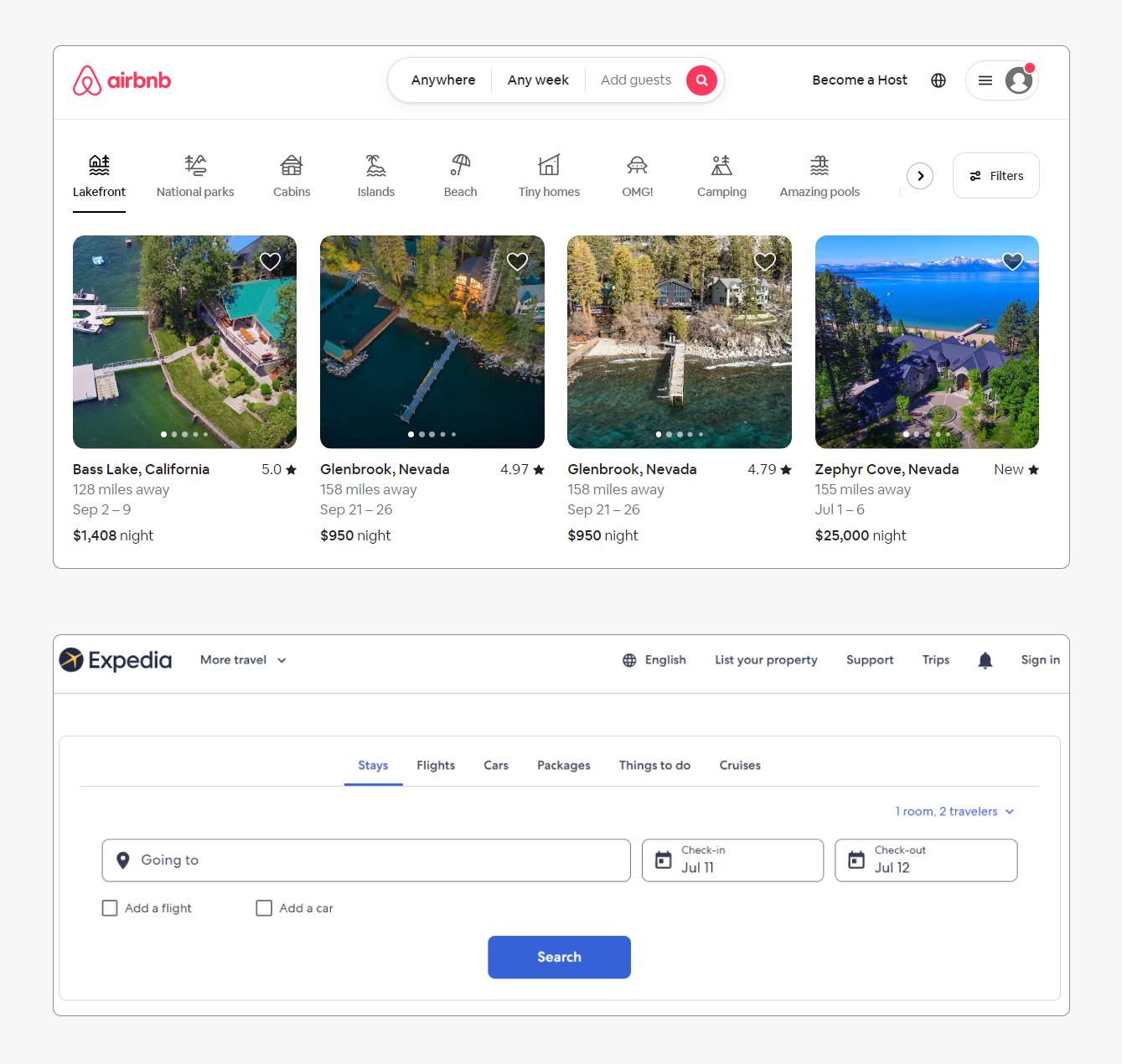The image is a screenshot of a travel web page, featuring two combined screenshots stacked vertically. The background is light gray, and each of the two pages is presented within a rectangular pane with rounded corners. These panes have a thin, medium gray outline and a white background.

**Top Pane:**
- **Header Section:**
    - On the left side of the header is a pink, A-shaped logo formed by a curly Q line.
    - Adjacent to the logo is pink lowercase text reading "Airbnb."
    - After some negative space to the right, there is a pill-shaped area with a medium gray outline, divided into three sections by thin separator lines:
        - The left section has bold black text stating "Anywhere."
        - The middle section reads "Any Week."
        - The right section, in light gray, says "Add Guests."
    - To the right of this search bar, there is a pink circle containing a white magnifying glass icon.
    - Further right, after some negative space, bold black text reads "Become a Host."
    - Next, there is a black gridded globe icon.
    - Finally, on the far right, a white pill-shaped icon with a thin medium gray outline contains:
        - A black hamburger menu on the left.
        - A medium gray circle on the right with a white profile picture icon, partially eclipsed by a pink dot on its upper right side.
- **Below the Header:**
    - A thin light gray line separates the header from the next row.
    - Underneath this line, there is a row of medium gray icons with accompanying medium gray labels.

This detailed description provides a clear visual representation of the travel web page screenshot as described.